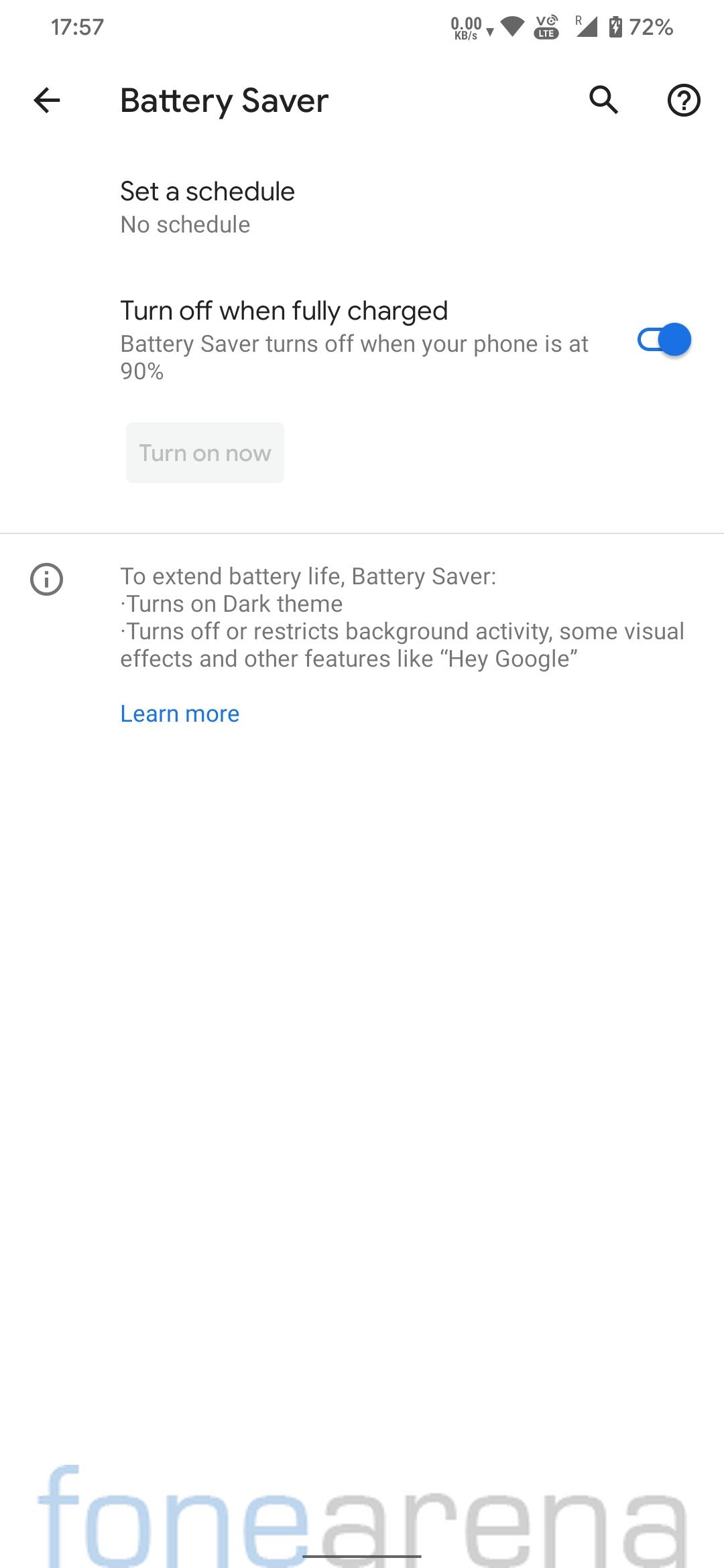Screenshot Description:
The image is a screenshot of a smartphone screen displaying the battery settings menu against an all-white background. 

**Top Status Bar:**
- The top-left corner shows the current time, 17:57.
- The top-right corner includes several icons:
  - "000" with a downward-pointing triangle, indicating some kind of dropdown menu.
  - A Wi-Fi symbol.
  - An LTE symbol.
  - A full-service signal bars indicator.
  - A battery icon showing a 72% charge.

**Battery Settings Menu:**
- The screen header has a back button, a battery saver toggle, a search icon, and a help icon (question mark).
- Below the header:
  - A section labeled “Set a schedule” that shows no schedule is set.
  - A toggle labeled “Turn off when fully charged,” which is enabled as indicated by its blue color. It mentions that the battery saver turns off when the phone reaches 90% charge.
  - A grayed-out button labeled "Turn on now," suggesting that battery saver is currently active.

**Information Section:**
- Below this, a description explains that to extend battery life, the battery saver enables a dark theme and restricts background activity, some visual effects, and other features, including Google services.
- A "Learn more" link is provided in blue text for additional information.

**Footer:**
- At the very bottom of the screen, the words "phone arena" appear, with "phone" styled as "f-o-n-e" in blue and "arena" in gray, both in light font.

This detailed description captures all the text and visual elements displayed in the screenshot of the battery settings menu on a smartphone screen.